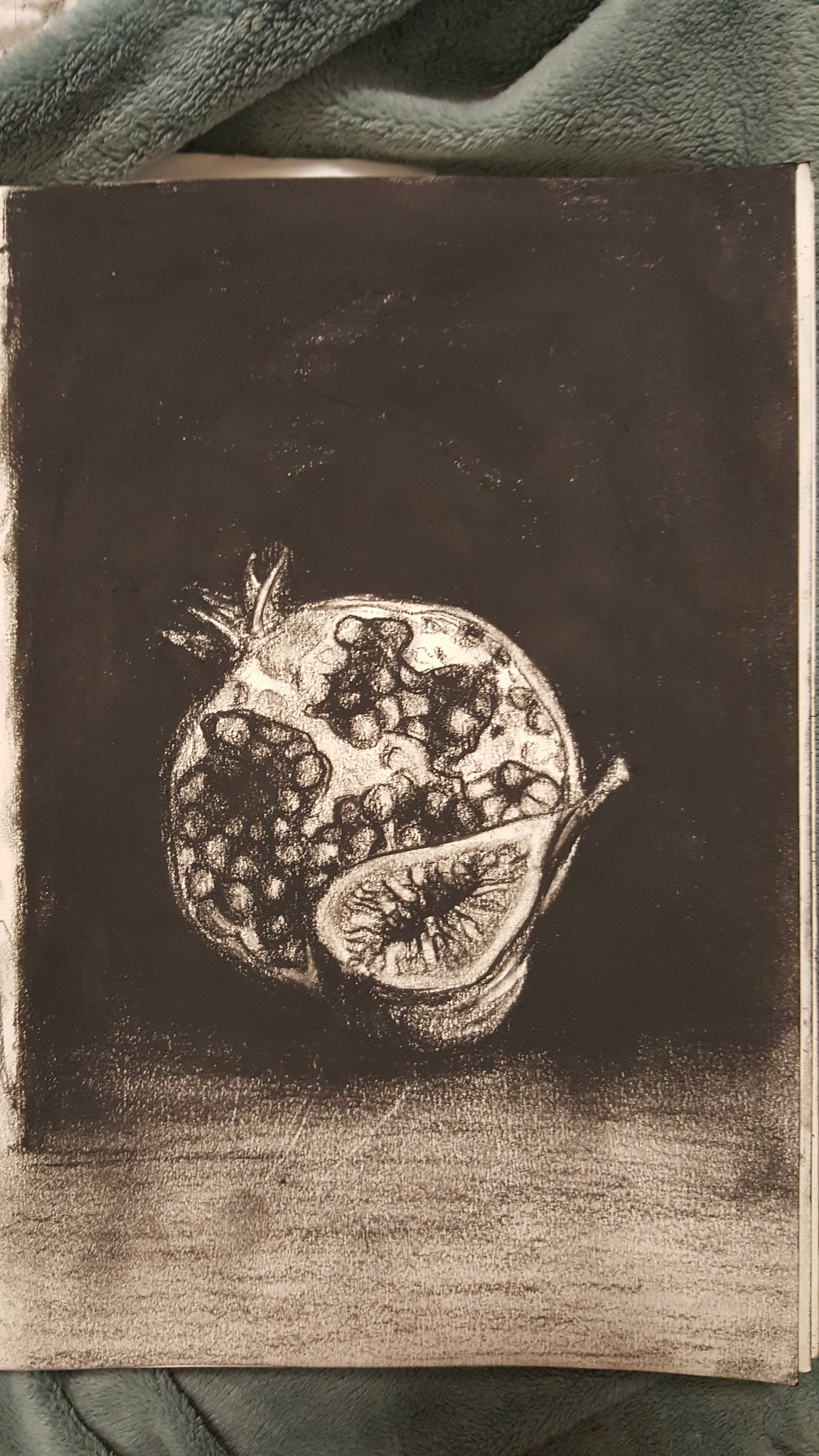An exquisitely detailed charcoal illustration captures a sectioned pomegranate, revealing its intricate interior. The exposed flesh, depicted in varying tones of white, contrasts sharply with the seeds, which are richly rendered in multiple shades of black and gray, showcasing their distinctive shapes and remnants. At the top left, a stem and a few leaves extend from the pomegranate, adding a touch of natural detail. In the bottom right of the composition, another plant, possibly a fruit with a teardrop shape, features a shadowed section within, hinting at its internal structure. This second plant also has a small stem protruding from its right side. The backdrop of the illustration consists of a dramatic black expanse at the top, transitioning to a gray area at the bottom, providing a stark contrast to the subjects. The entire scene is set upon a textured, greenish towel or blanket, grounding the composition with a touch of color amid the monochromatic subject matter.